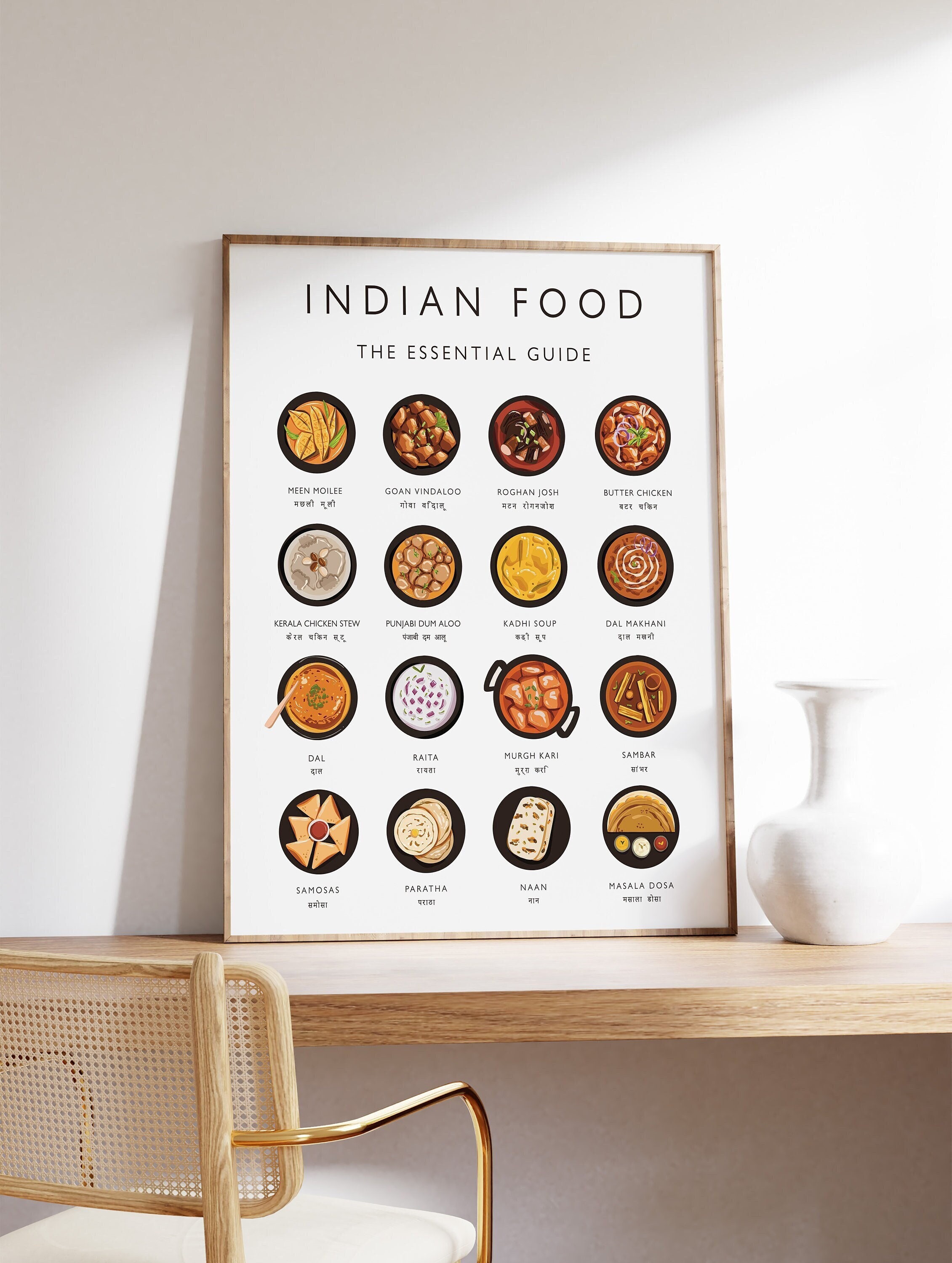The image showcases a detailed interior scene centered around a wooden half-table propped against a white wall. On the table, there is a prominently displayed poster framed in wood that reads "Indian Food, The Essential Guide." The poster is positioned in the center of the table and features 16 circular images, each depicting a different Indian dish, with names written beneath each picture. The dishes include an assortment of curries, soups, breads, and side dishes, all contained within round pots. The background of the poster is white and the text is in black, emphasizing the colorful images of the food. To the bottom left of the table, there is a gold and wooden chair with a woven rattan back and a white cushion, matching the white vase placed just in front of the desk to the right of the poster. The overall design is minimalistic, enhancing the presentation of the Indian dishes.